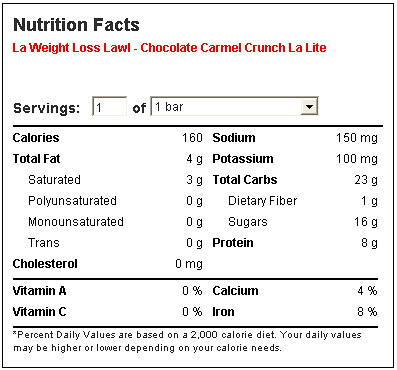A close-up image showcases the intricate details of a nutrition label for a chocolate caramel crunch bar produced by Law's Laurel. The label, resembling a digital interface possibly displayed on a computer screen, indicates comprehensive nutritional information for a single serving, which is one bar. Key nutritional details include 160 calories, 4 grams of total fat, broken down into 3 grams of saturated fat, and zero grams each of polyunsaturated, monounsaturated, and trans fats. The bar contains no cholesterol, 150 milligrams of sodium, 100 milligrams of potassium, 23 grams of total carbohydrates (including 1 gram of dietary fiber and 16 grams of sugar), and provides 8 grams of protein. The dropdown menu suggests a feature allowing for the selection of a variable number of bars, tailoring the nutritional information accordingly. The light appears low, emphasizing the text on the label, with clear visibility of all components.